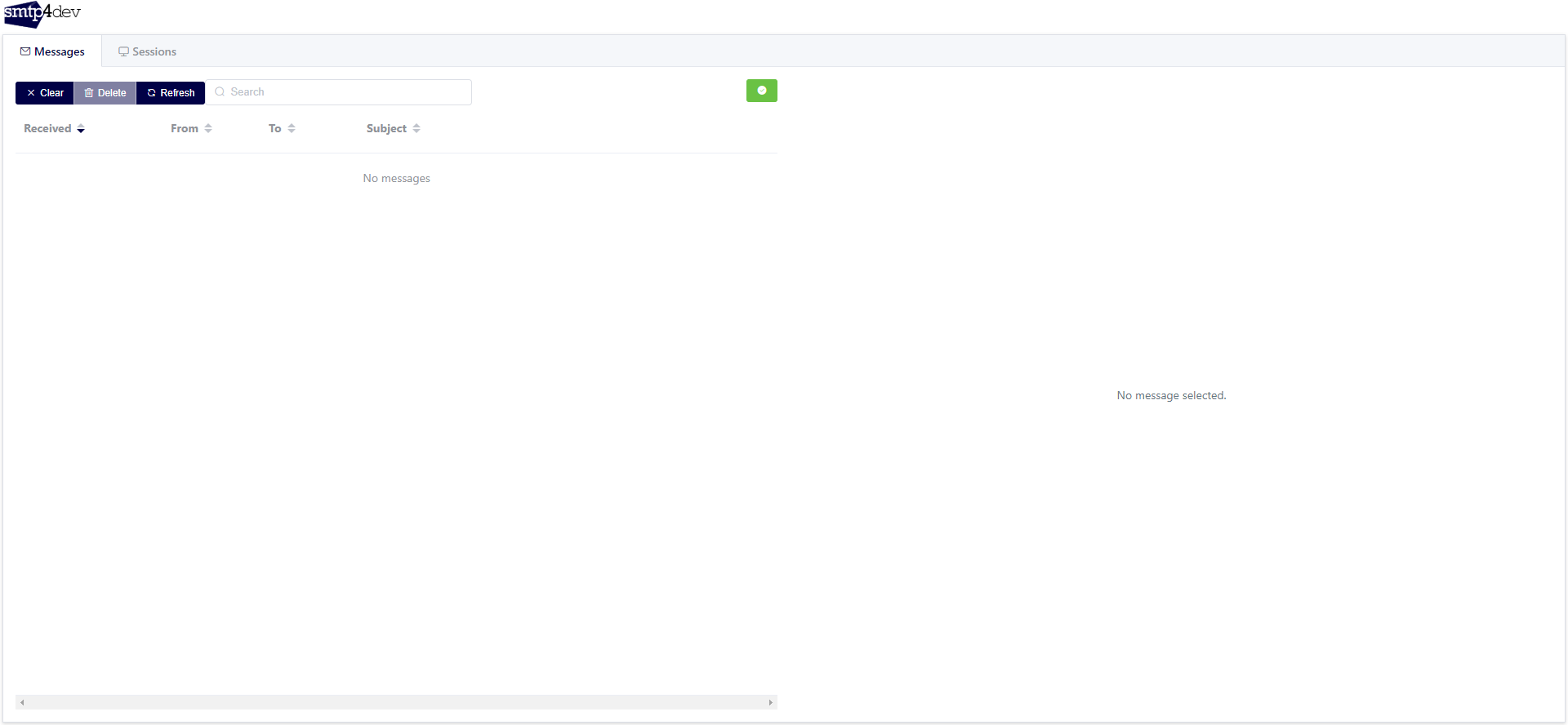The website features a minimalist design with an emphasis on white space. In the upper left corner, the site prominently displays the text "SMTP4DV." The "SMTP" segment is placed on a blue, geometric, pentagon-like shape, making the letters white, while "4DV" is styled in black. 

Below this header, there are two main tabs labeled "Messages" and "Sessions," with "Messages" currently being the active tab. Directly beneath the tabs, three buttons are aligned horizontally: "Clear" in navy blue, "Delete" in gray, and "Refresh" also in navy blue. All button labels are displayed in white, reverse print.

To the right of these buttons is a search bar, centrally positioned within the page's layout. Additionally, a green square with a white dot appears adjacent to the search bar, its function unclear.

Further down, the interface presents columns labeled "Received" (with a downward-pointing arrow), "From," "To," and "Subject." Currently, the message area is empty, displaying "No messages." In the same central-right alignment, "No message selected" is reiterated.

At the bottom of the page, a gray taskbar allows horizontal navigation, indicating additional content width beyond the visible area. Scrolling left or right using this taskbar may reveal more of the page's interface.